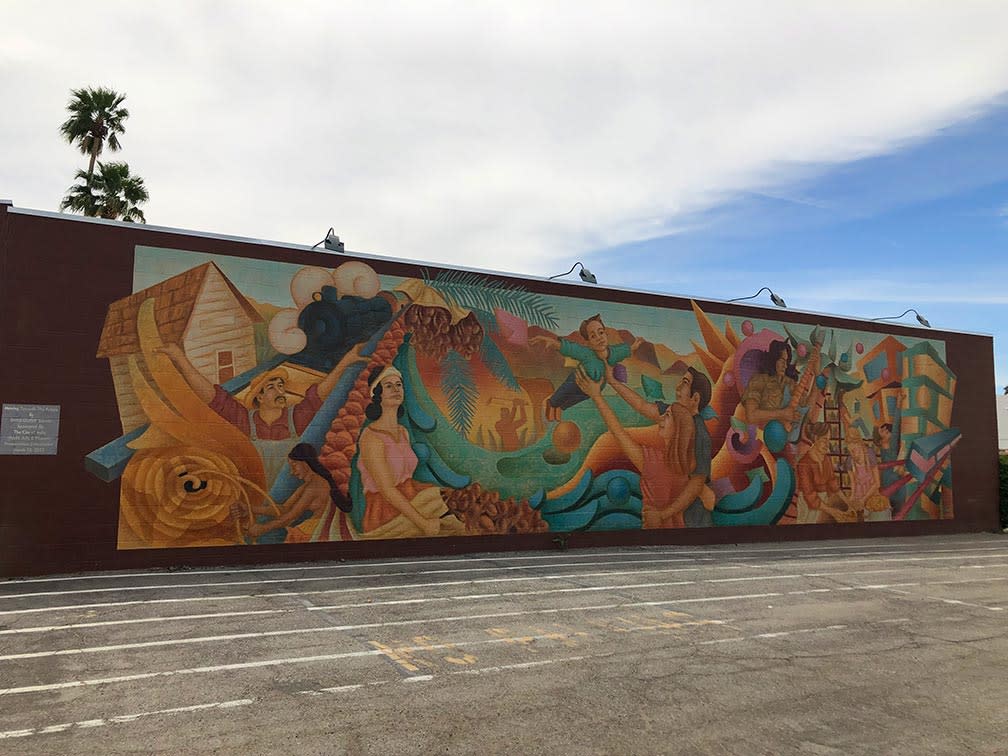The image depicts an expansive, vibrant mural on the exterior wall of a one-story red brick building. This vertically oriented mural, richly colored in vivid teals, purples, blues, and golds, covers most of the building's façade, which sits alongside a well-maintained sidewalk.

The mural's theme appears to celebrate Latino culture and labor. At the heart of the mural is a farm worker, a man wearing overalls with his arms outstretched, standing against a backdrop that includes a house and a train, suggesting a journey or a connection between rural and urban life. Various workers are depicted, including a woman carrying a large bag of what looks like cocoa or coffee beans, symbolizing agricultural labor. 

There are also grapes or a fruit-like substance featured prominently, highlighting the agricultural abundance. Additionally, a modern couple is present, cradling a child who plays airplane with outstretched arms, symbolizing hope and future generations. The mural also incorporates images of futuristic homes and diverse characters, tying together past, present, and future within the Latino community.

The scene is set under a bright blue sky dotted with clouds, and a palm tree can be seen in the background, adding to the overall vibrant and lively atmosphere captured in the mural.